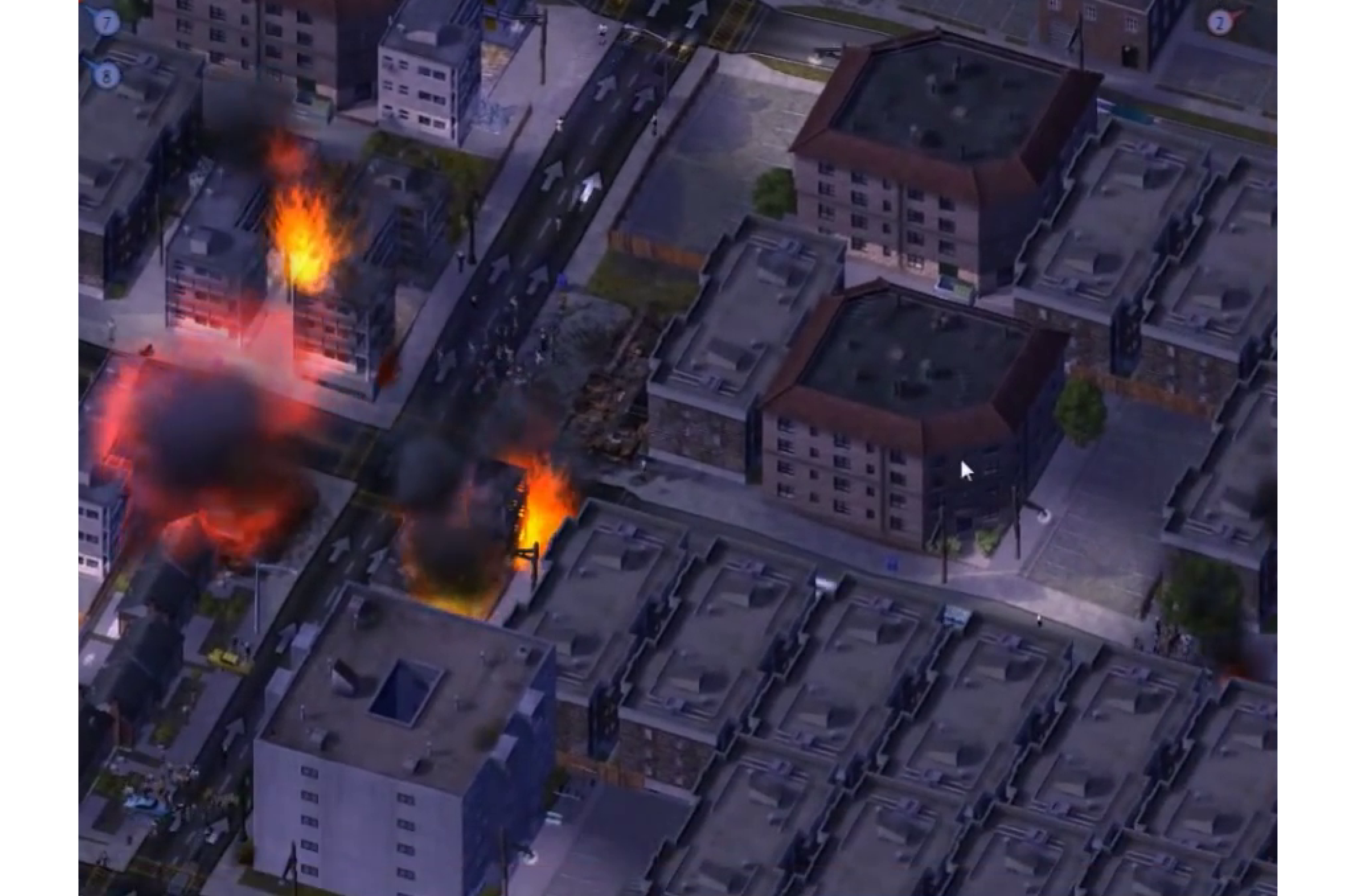This aerial nighttime image presents a cityscape that appears digitally rendered, reminiscent of a video game. The scene primarily features clustered, low-rise buildings around four or five stories high, all depicted in varying shades of gray. The layout includes rooftops, plots of space resembling parking lots, and a roadway running from the bottom left to the middle top of the image. On the left side, attention is drawn to three buildings engulfed in vivid red, orange, and yellow flames, emitting gray and black smoke. Tiny figures are visible on the streets below, though their activities are indiscernible. The overall lack of fine detail in the buildings and the digitized appearance lend the image an almost surreal, artificial quality.